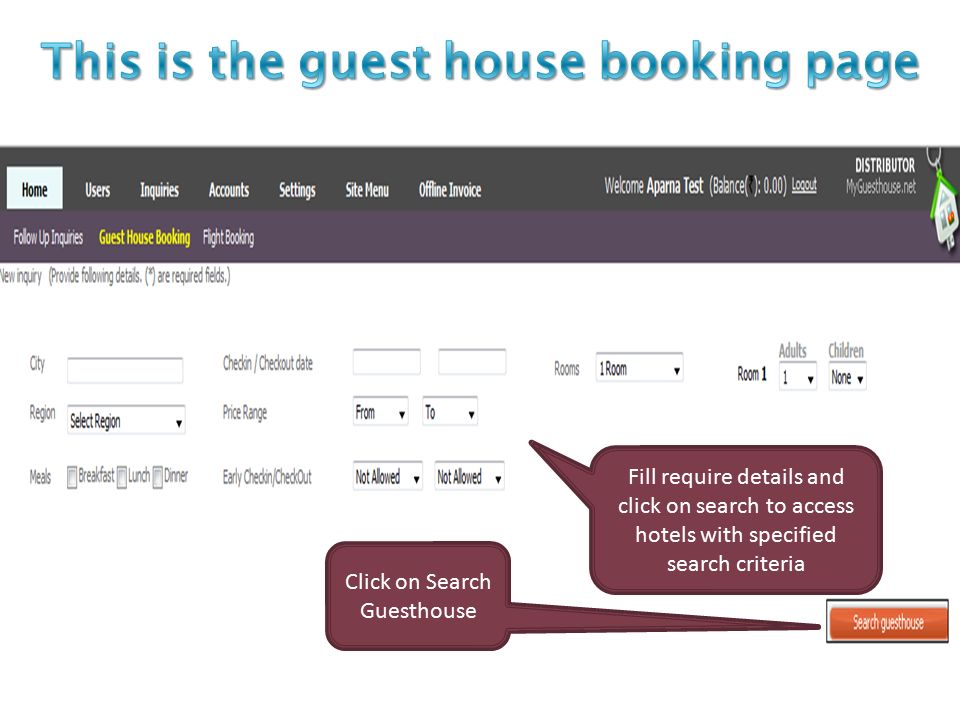This image depicts the homepage of a website, myguesthouse.net, specifically the guesthouse booking page. At the very top, there is a prominent turquoise blue text header indicating "This is the guesthouse booking page." Beneath this, a clean white space leads to a horizontally long, rectangular box.

The upper half of this box features a black ribbon containing navigational options from left to right: Users, Inquiries, Accounts, Settings, Site Menu, and Offline Invoice. Towards the right of this ribbon are the options: Welcome, A PAMA Test, Balance (with zeros in parentheses), and Logout (underlined). Below this black ribbon, in bold white text, the word "Distributor" is displayed, followed by "myguesthouse.net" underneath.

Adjacent to these elements, there is a small image of a white house with a green roof, resembling a keychain. To the far left of this section, the word "Home" appears prominently highlighted inside a white box.

Beneath the black ribbon, a purple section extends horizontally, displaying the options Follow-up Inquiries, Guesthouse Booking, and Flight Booking in white text. Among these, "Guesthouse Booking" is distinctly highlighted in yellow, indicating it as the current page or selection.